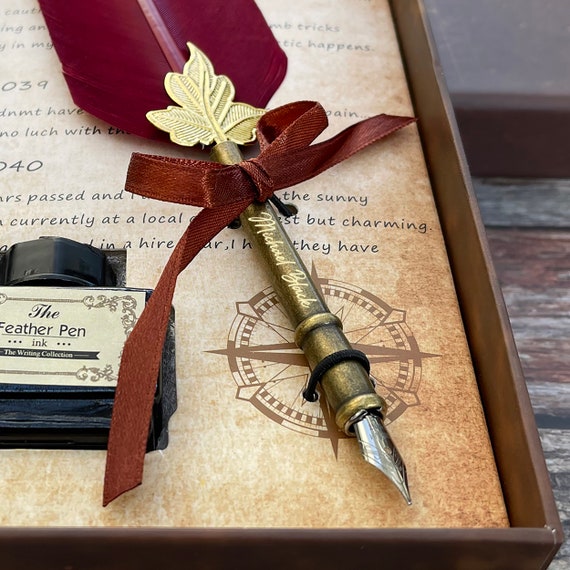This photograph features a nostalgic, framed display of a vintage-style feather pen set, meticulously arranged on a weathered wooden table. At the center is a brown feather pen adorned with a maroon feather and a maroon ribbon tied around its shaft. The pen's casing proudly displays the engraved name "Michael Black" in gold lettering, with a gold leaf charm positioned at the base of the feather, and a sharp silver tip designed for writing. The pen is secured to a parchment-style paper within the brown gift box, which bears additional text and intricate prints, including a compass motif. To the left of the pen is a card with the inscription "The Feather Pen Ink, The Writing Collection," hinting at the bottle of ink that accompanies the set. This elegant composition, evoking a sense of old-world charm, is carefully framed and primarily showcases a harmonious blend of brown and gold tones.